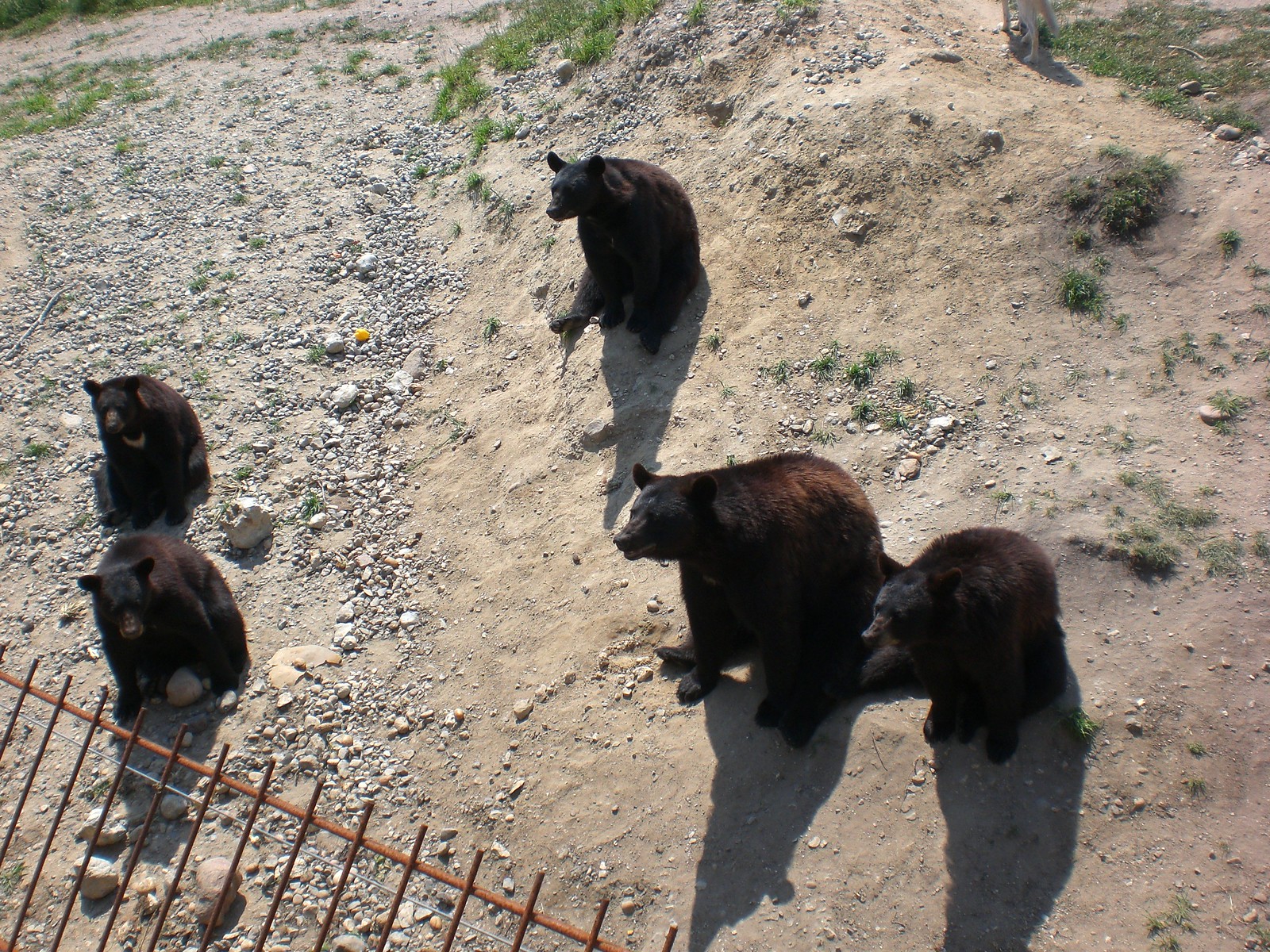This is a detailed color photograph taken at a zoo, showing five brown bears in an enclosure. The enclosure features a light brown, rocky ground with small stones scattered throughout and sparse areas of green grass in the background. The bears, with darker brown faces and ears, exhibit varying sizes; three smaller cubs are situated to the left, while two larger bears, possibly the parents, are positioned to the right. Most of the bears appear to be gazing towards the left side of the frame with an almost bored demeanor. A thin, rust-colored wrought iron fence separates the viewers from the bears, partially fallen over to the bottom left of the image. In the upper part of the background, the faint legs of another animal, likely white, can be seen but are not clearly identifiable. The sunlight casts a reddish-brown tint on the bears' fur, adding a rich contrast to their otherwise dark brown coats.